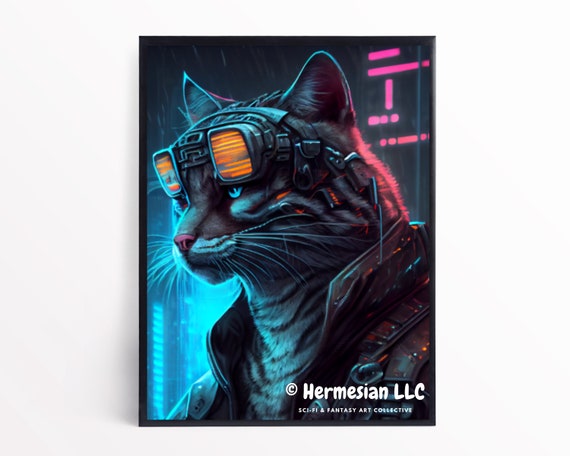The image features an intriguing gray cat with black stripes, set against a striking black and blue backdrop. The cat exudes a futuristic vibe with robotic elements integrated into its appearance, particularly a set of advanced-looking glasses connected by wires that run down the sides of its head. Its piercing blue eyes are accentuated by the glow of a neon blue light shining upon it, enhancing its somewhat cybernetic aura. In the background, the words "Hermesian LLC" appear in white, accompanied by the phrase "Sci-Fi and Fantasy Art Collective." Additionally, pink neon lights are visible, illuminating what appears to be a large building, adding depth and further emphasizing the sci-fi theme. The overall effect captures the essence of a cool and captivating feline in a high-tech, fantastical setting.